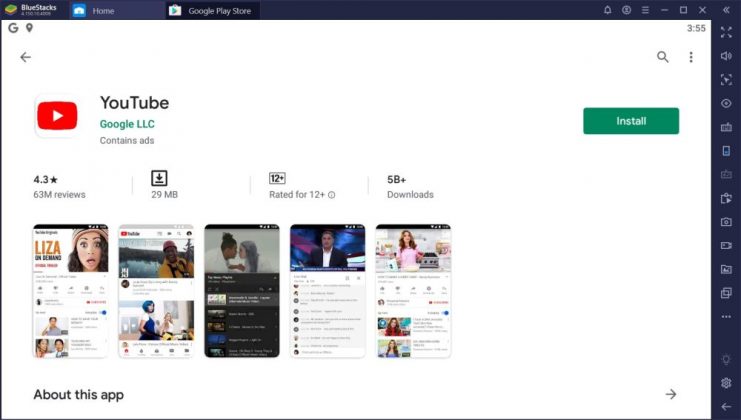The screenshot displays the BlueStack interface. At the top left corner, the BlueStack logo is visible with an illegible text underneath it. Moving right from the logo are the navigation options: "Home", "Google Play Store" in the center, and on the far right, icon buttons for Notifications (bell), User Profile, Menu (three stacked lines), Minimize, Maximize, and Close. Additionally, a figure of $3.55 is displayed.

Beneath this, the main content of the screen is predominantly white featuring details of the YouTube app by Google LLC. At the top, there's a Google 'G' icon, a pushpin icon, and a left-facing arrow. The header "YouTube" is in bold black next to its icon - a red button with a white play symbol. Below this, the text "contains ads" is noted, with "Install" prominently displayed in a green button on the right.

The app details include a star rating of 4.3 based on 63 million reviews, total downloads of 29 million, an age rating of 12+, and an indicator showing 58+ downloads. To depict the app, there are five thumbnail images of cell phone screens, showcasing various aspects of YouTube. Towards the bottom of the screen, there is a section titled "About this app."

The page's overall color scheme includes white, red, green, blue, pink, orange, and yellow accents.